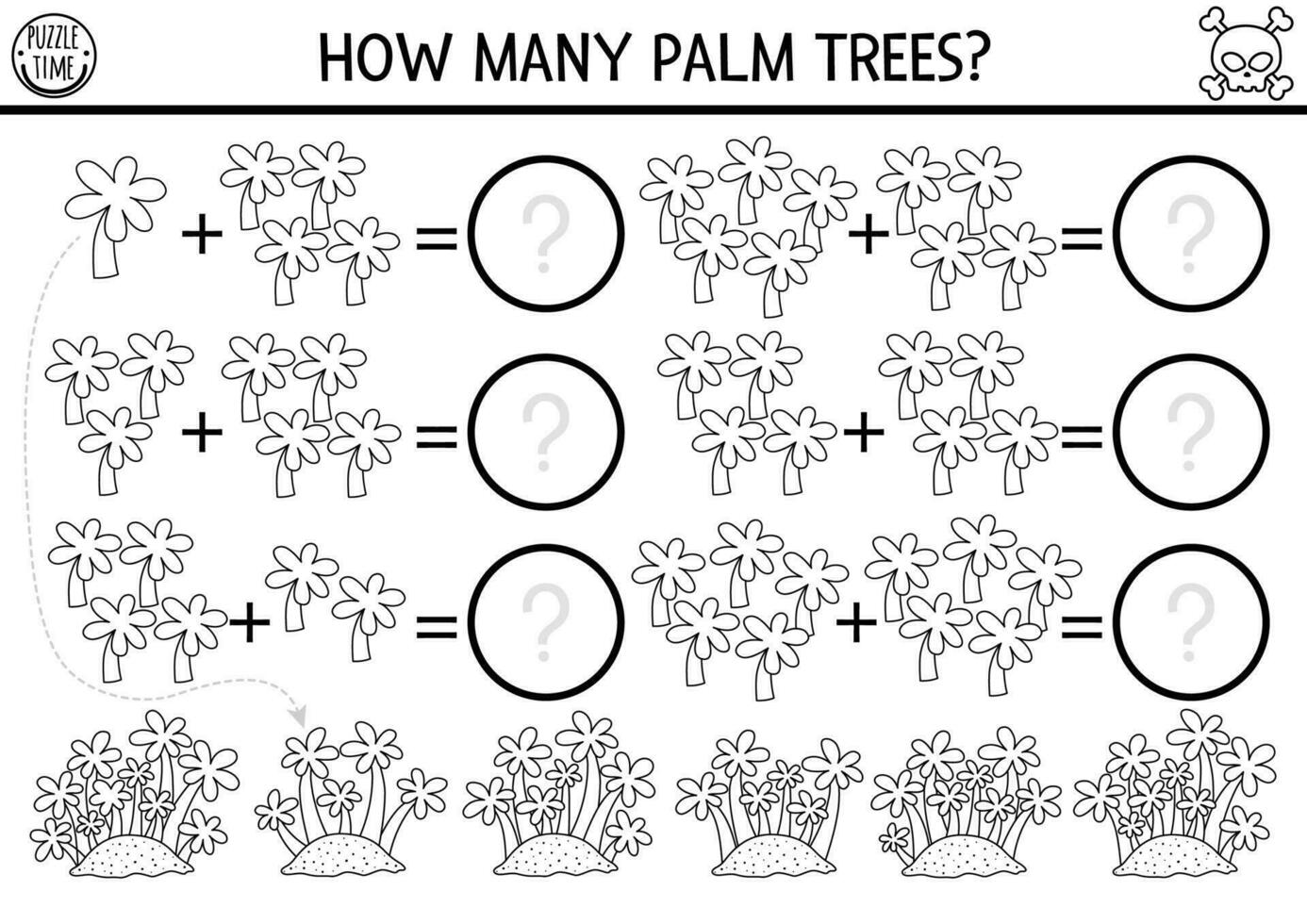This image is a black and white worksheet designed for elementary school children to practice addition with a fun theme. At the top of the page, bold text asks "How Many Palm Trees?" accompanied by a question mark. On the upper left-hand corner, the words "Puzzle Time" appear with a smiley face, while the upper right-hand corner features a skull and crossbones.

The worksheet is structured to engage children through visual puzzles. Each row begins with a simple addition problem involving palm trees drawn in a sketchy style. The first equation shows one palm tree plus four palm trees, which equals a circle with a question mark in the center, prompting students to solve the sum. Each subsequent row increases the numbers being added, for example, three palm trees plus four palm trees.

Arrows guide the children from these equations to a section at the bottom of the page, labeled "Palm Tree Island," where various clusters of palm trees are illustrated. The aim is for children to match the sum from each row to the corresponding group of palm trees on the island. The worksheet is both educational and visual, making addition engaging and accessible for young learners.